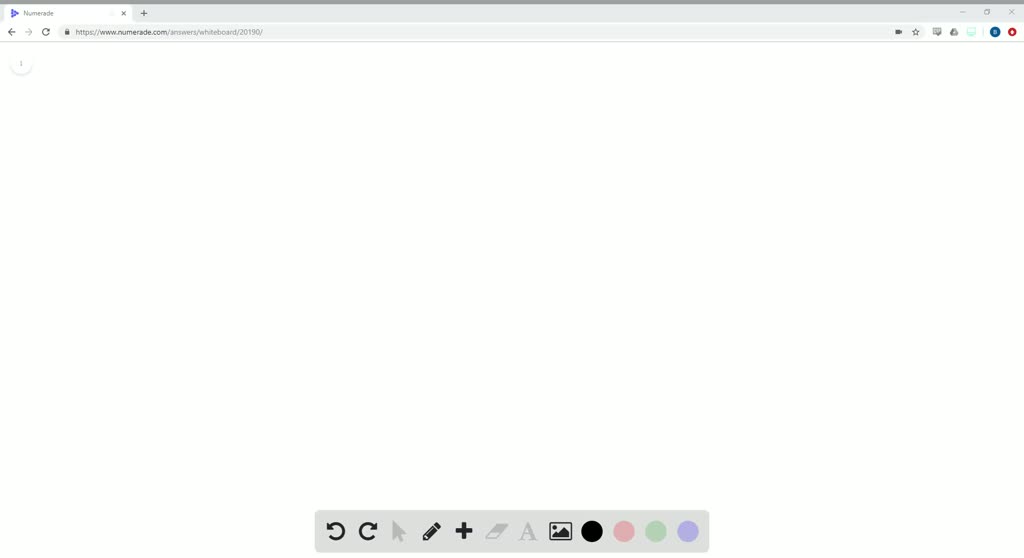The image depicts a minimalist and largely uncluttered user interface (UI) of a web browser. In the top left corner, there is a single browser tab, positioned directly above a search bar. To the right of these elements, there are six small icons, although they are barely discernible due to the zoomed-out perspective of the image. 

On the top right corner of the browser window, there are three standard window control buttons: minimize, maximize, and close.

The remainder of the interface features a white background. Along the bottom, there is a grey rectangular toolbar containing several tabs and icons. From left to right, these icons include two refresh buttons, an arrow, an editing icon, a plus icon, two grey icons, followed by a gallery icon, a black circle, a pink circle, a green circle, and a purple circle.

Overall, the image showcases a sparse and clean browser layout, with a focused selection of functional icons available for user interaction at the bottom of the window.